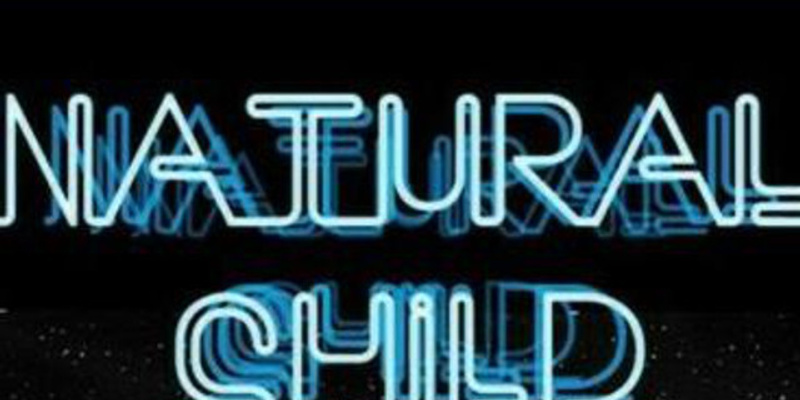In the image, a sign reading "NATURAL CHILD" is displayed against a predominantly black background. The sign's letters, which appear to be crafted from neon tubes, emit a striking blue glow. The word "NATURAL" is positioned above the word "CHILD," both capitalized and spaced closely together. The design incorporates a clever visual effect where the letters of both words are repeated multiple times in the background, transitioning from white to lighter blue and finally to a darker blue. This repetition creates a compelling 3D, retro appearance, reminiscent of neon signs on buildings. Additionally, there's a slightly visible, vague texture beneath the words that looks like an asphalt road with tiny white specks, adding to the image’s depth. The top and side portions of the word "NATURAL" and the lower part of "CHILD" appear slightly cropped, suggesting a close-up view. The far background contains indistinct, blurry lights, which might be city lights, enhancing the nocturnal ambiance.